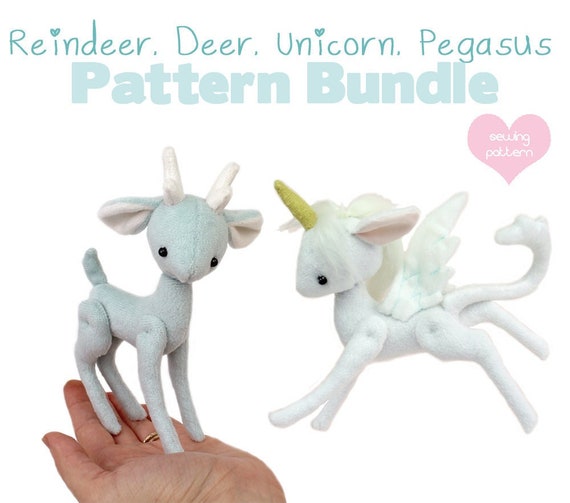A whimsical photograph showcases two small, thin stuffed animals that look perfect for a young child. The image features a gray deer with horns and a short tail, standing beside a gray unicorn with a single yellow horn, white wings, and a long tail that ends in a small head-like shape. The ears of both animals are a very light pink and white. The top of the image has a playful, kid-friendly font that reads "Reindeer, Deer, Unicorn, Pegasus" with each letter 'i' dotted with a heart. Above this text, the words "Pattern Bundle" are prominently displayed in a larger, light teal sans-serif font. A pink heart with the words "Sewing Pattern" is also visible near the unicorn. One of the stuffed animals is held in a hand, showing their small size, perfect for fitting into a child's palm.